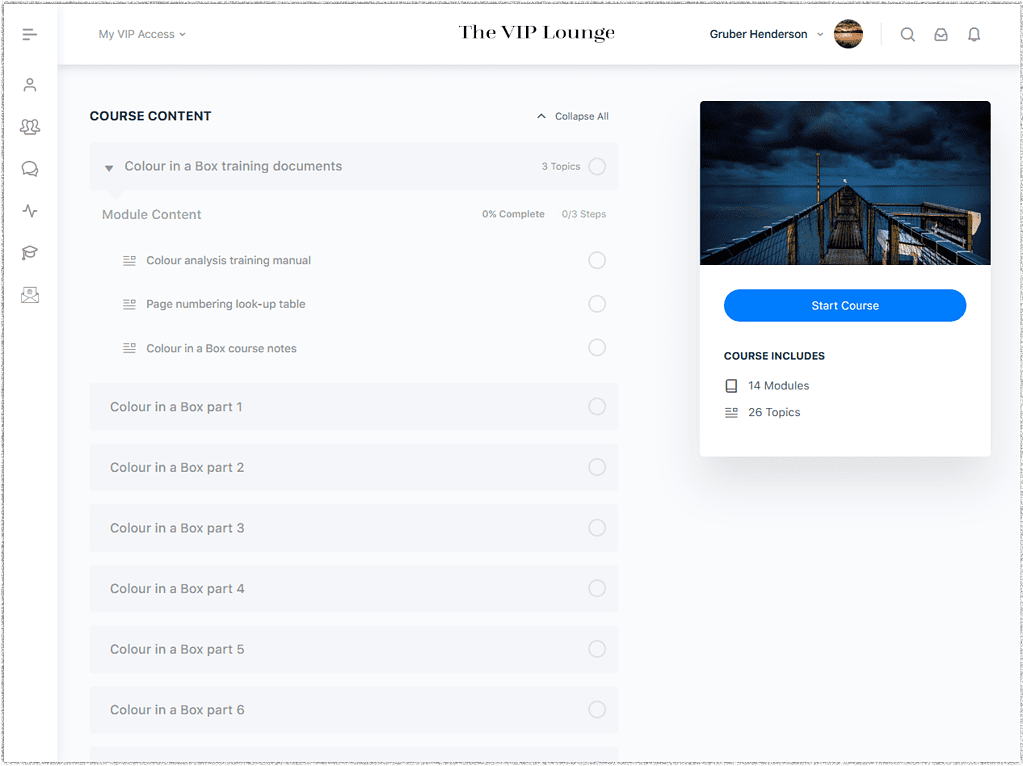In this photo, an opened software on a computer screen is displayed. At the very top of the screen, the title "My VIP Access" appears with a small drop-down arrow beside it. Centered at the top is the name of the software website, "VIP Lounge." Moving toward the right-hand side, the user's name, "Gruber Henderson," is displayed in dark blue alongside a drop-down arrow and a profile picture. Adjacent to these elements are three small icons: a search icon, a mail icon, and an alert icon.

Running vertically along the left-hand side of the screen is a menu featuring six icons, each representing different sections of the software. The current page focuses on course content, with an option at the top to collapse or expand all sections. This page is fully expanded.

The featured course is “Color-in-a-Box Training Documents,” with its content divided into distinct modules: Color-in-a-Box Part One, Part Two, Part Three, Part Four, Part Five, and Part Six. Each module is contained within gray rectangles that can be selected to reveal additional options.

On the right-hand side of the screen, there is a scenic photo. Below this image, a button labeled "Start Course" is visible, noting that the course includes 14 modules and 26 topics.